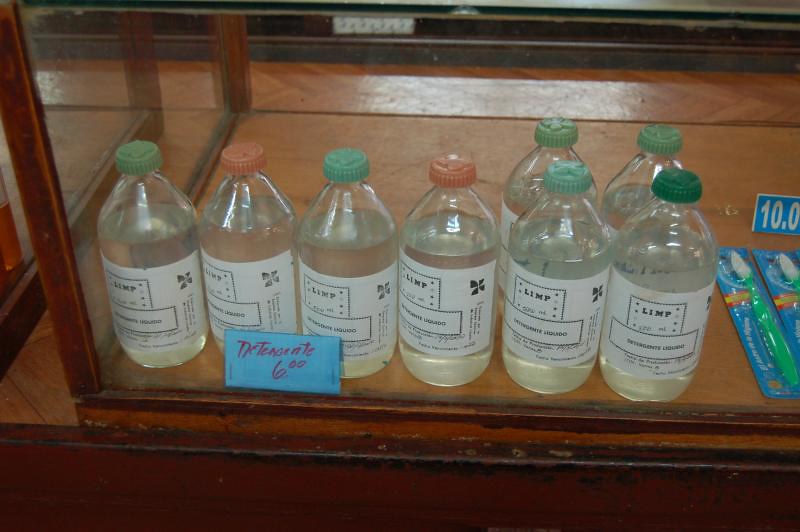This image depicts an older pharmacy display counter made of plain brown wood with a glass pane showcasing various items for sale. Behind the glass, there are eight bottles arranged in a row from left to right, all featuring a uniform white label with legible black text reading "LIMP" at the top center. The bottles contain a clear liquid and are capped with either green or orange tops; specifically, six have green caps while two have orange caps. In front of these bottles, there is a small blue card displaying a handwritten note that reads "600," likely indicating the price, along with possibly the name of the item, though it is barely legible—suggested words include "Detente" or "Detensate." To the right side of the counter, there are packaged toothbrushes with green handles and white heads, encased in blue packaging. Additionally, a blue sign behind the toothbrushes appears to read "10.0," though it is partially obscured.